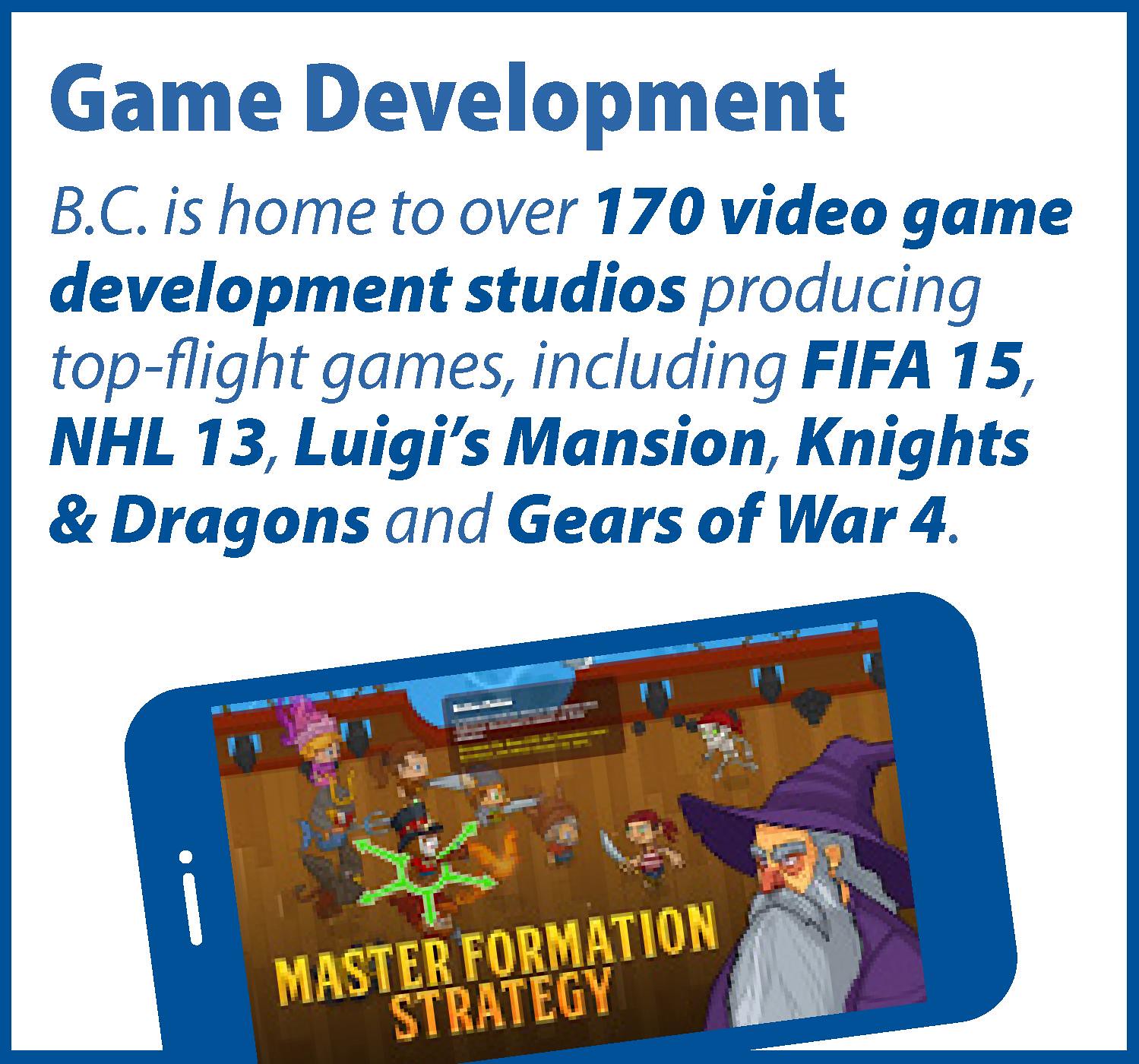The image is a graphic advertisement designed with a blue border and white background, featuring the heading "Game Development" in blue. The text below reads: "BC is home to over 170 video game development studios, producing top-flight games including FIFA 15, NHL 13, Luigi's Mansion, Knights & Dragons, and Gears of War 4," with important elements like "170 Video Game Development Studios" and the game titles highlighted in bold.

Central to the image is an illustration of a blue iPhone tilted sideways. On the iPhone screen, there is a pixelated game depicting a wizard with a long gray beard, purple wizard's hat, and cloak, located in the lower right-hand corner. Alongside the wizard, various characters are shown, including a pirate wearing a red and white shirt and headscarf, holding a sword; an animal sporting a top hat; and a skeleton adorned with a red headdress. The background includes a pirate ship and water, enhancing the adventurous theme. In pixelated yellow text at the lower left-hand corner of the phone screen, the words "Master Formation Strategy" are visible.